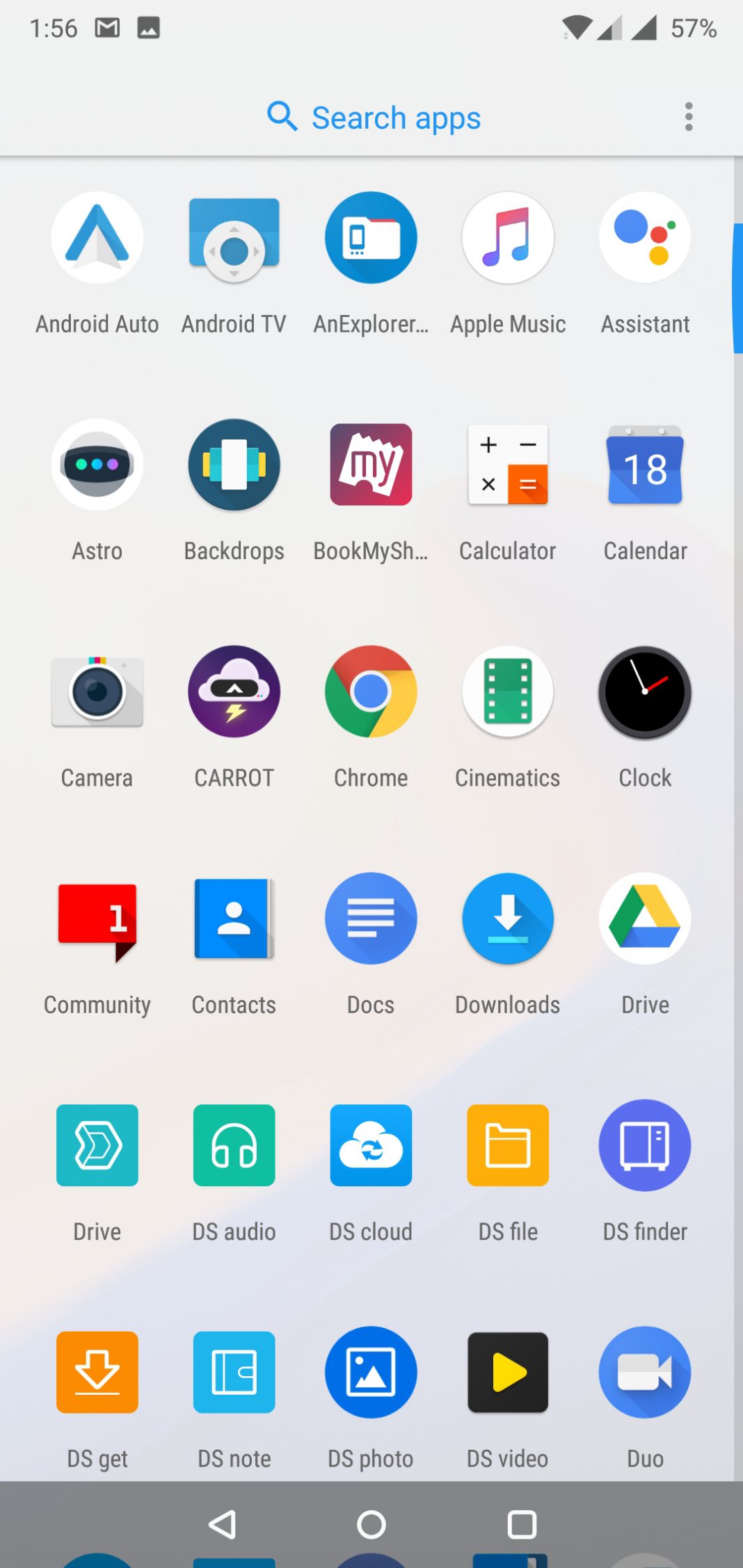This is a detailed screenshot of a smartphone displaying a portion of its apps. At the top of the screen, there is a horizontal status bar showing "156" on the left. To the right of this number, there is the Google email icon followed by the gallery icon for the camera. On the far right side of the status bar, there is a series of connectivity and battery indicators: fully connected Wi-Fi symbol, a set of bars showing half signal strength, another set of bars indicating full service strength, and finally, the battery percentage at 57%.

Below the status bar, there's a "Search apps" field highlighted in light blue, with three vertical dots positioned on the right side of this bar.

The main section of the screenshot showcases some of the installed apps organized in rows of five. The visible list of apps includes:

- Row 1: Android Auto, Android TV, Explore, Apple Music, Assistant
- Row 2: Astro, Backdrops, BookMyShow, Calculator, Calendar
- Row 3: Camera, Carrot, Chrome, Cinematics, Clock
- Row 4: Community, Contacts, Docs, Downloads, Drive
- Row 5: Drive, DS Audio, DS Cloud, DS File, DS Finder
- Row 6: DS Get, DS Note, DS Photo, DS Video, Duo

Each app is represented by its respective icon, making it easy to identify at a glance.